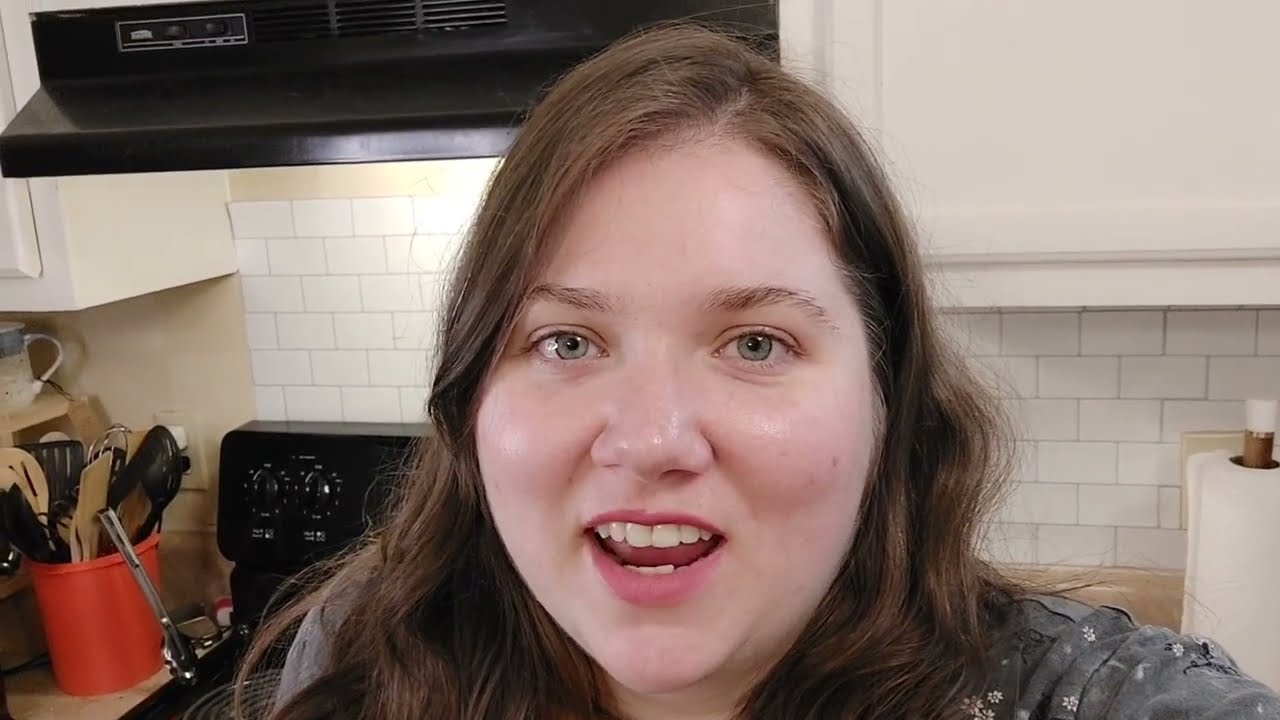In this selfie-style photograph, a Caucasian woman in her early 30s stands in her kitchen, close to the camera. She has pale skin, blue-gray eyes, and long brown wavy hair that cascades past her shoulders. Her face, which appears chubby with round cheeks, is prominently featured, and she seems to be caught mid-speech, revealing both rows of her teeth and her tongue.

She is wearing a gray shirt adorned with small daisy flowers. In the background, her kitchen features a backsplash of old white tiles with gray grout, a black stove with visible electric coils and a frying pan, a black vent hood, and various kitchen items. To her right, there’s a paper towel holder with a roll of paper towels, and to her left, an orange Rubbermaid container filled with kitchen utensils such as spatulas, wooden spoons, and ladles. The overall color scheme of the kitchen includes white, red, black, and gray tones.